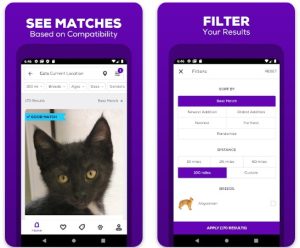The image comprises two screenshots from an animal adoption website designed to match potential pet owners with compatible animals.

- **Left Screenshot:** This side features a purple border with the text "See matches based on compatibility." Below this, search options are provided. The site displays a match, showcasing a black kitten with a white chest and striking yellow eyes. Additional options allow users to add the animal to their favorites, among other actions.
  
- **Right Screenshot:** This section also has a purple border and is labeled "Filter your results." It contains a white box similar in size to the one on the left. Here, users can select various filters to refine their search, including options to choose between dogs and cats. Due to the image's small and blurry nature, further details are difficult to discern.

Overall, the screenshots emphasize user-friendly features for finding a compatible pet through search options and filters, enhanced by a clear and attractive design.